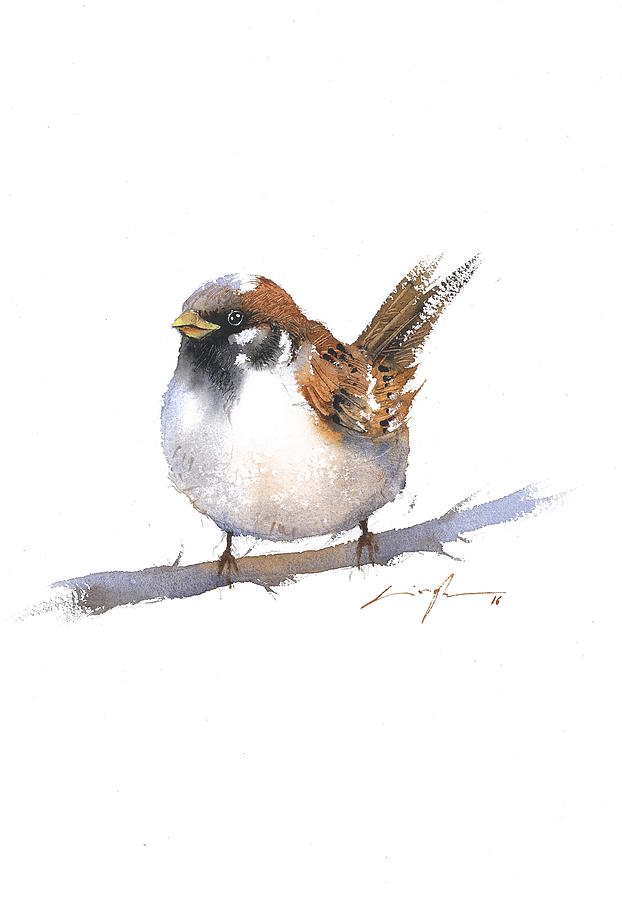This is a detailed watercolor painting of a small bird, likely a sparrow, perched on a branch against a stark white background. The bird is depicted with exquisite detail: its yellow beak stands out against its black face and throat, while its beady black eyes add a touch of liveliness. The top of its head is white, contrasting with brown feathers that extend from the back of its neck to its rump. Its wings and tail feathers are an intricate mix of browns, blacks, and whites, giving a speckled appearance. The bird’s round, chubby body and white chest emphasize its endearing form as it clutches the branch with tiny brown feet. The branch itself is rendered in varying shades of bluish-gray and medium brown, running horizontally across the image. The artist’s signature, difficult to decipher, is located beneath the right side of the branch, accompanied by the number '16' in brown. Overall, this well-executed piece beautifully captures the essence of the bird and its tranquil perch.